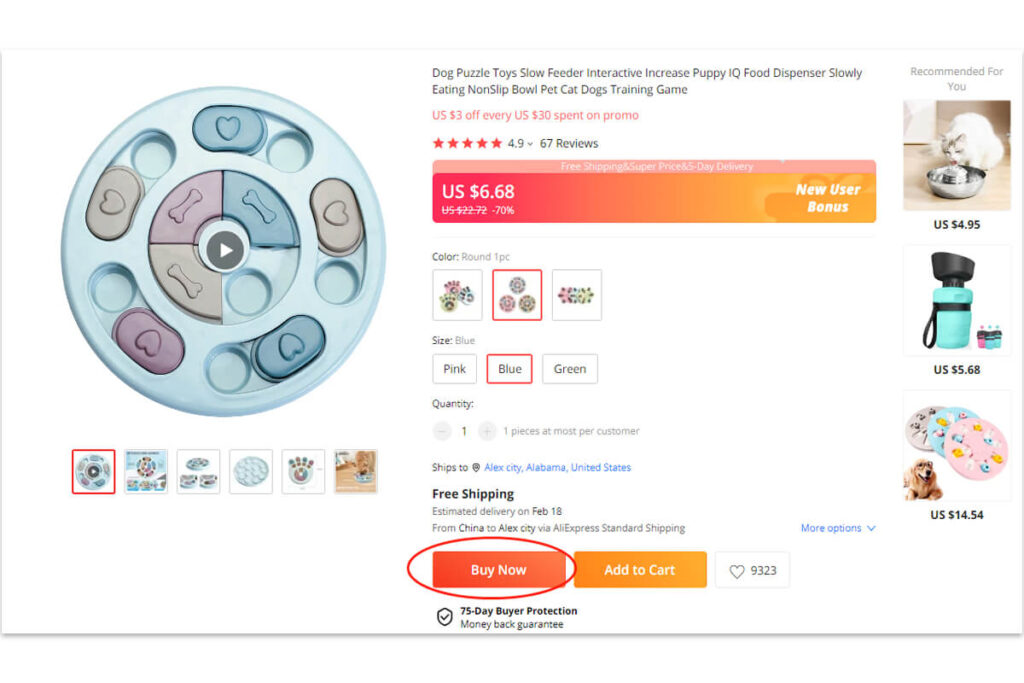The image showcases a promotional offer for a pet product titled, "Dog Puzzle Toys Slow Feeder." This interactive food dispenser is designed to increase a puppy's IQ and ensure they eat slowly, preventing non-stop consumption. The product caters to both dogs and cats, supporting their training and mental stimulation.

Highlighted in pink, the image advertises a special promotion: "US $3 off every US $30 spent." The product has received an impressive rating of 4.9 stars from 67 reviews and is available with free shipping. The price is marked down to US $6.68 from its original price of US $22.72, a significant 70% discount, with no additional user bonuses.

The quantity listed for purchase is one unit, scheduled to ship to a location in Alabama, United States. The estimated delivery date is February 18th, and the product will be shipped from China. 

At the bottom of the image, there's a rectangular, red "Buy Now" button, encircled with an oval-shaped red outline, inviting the user to make an immediate purchase.